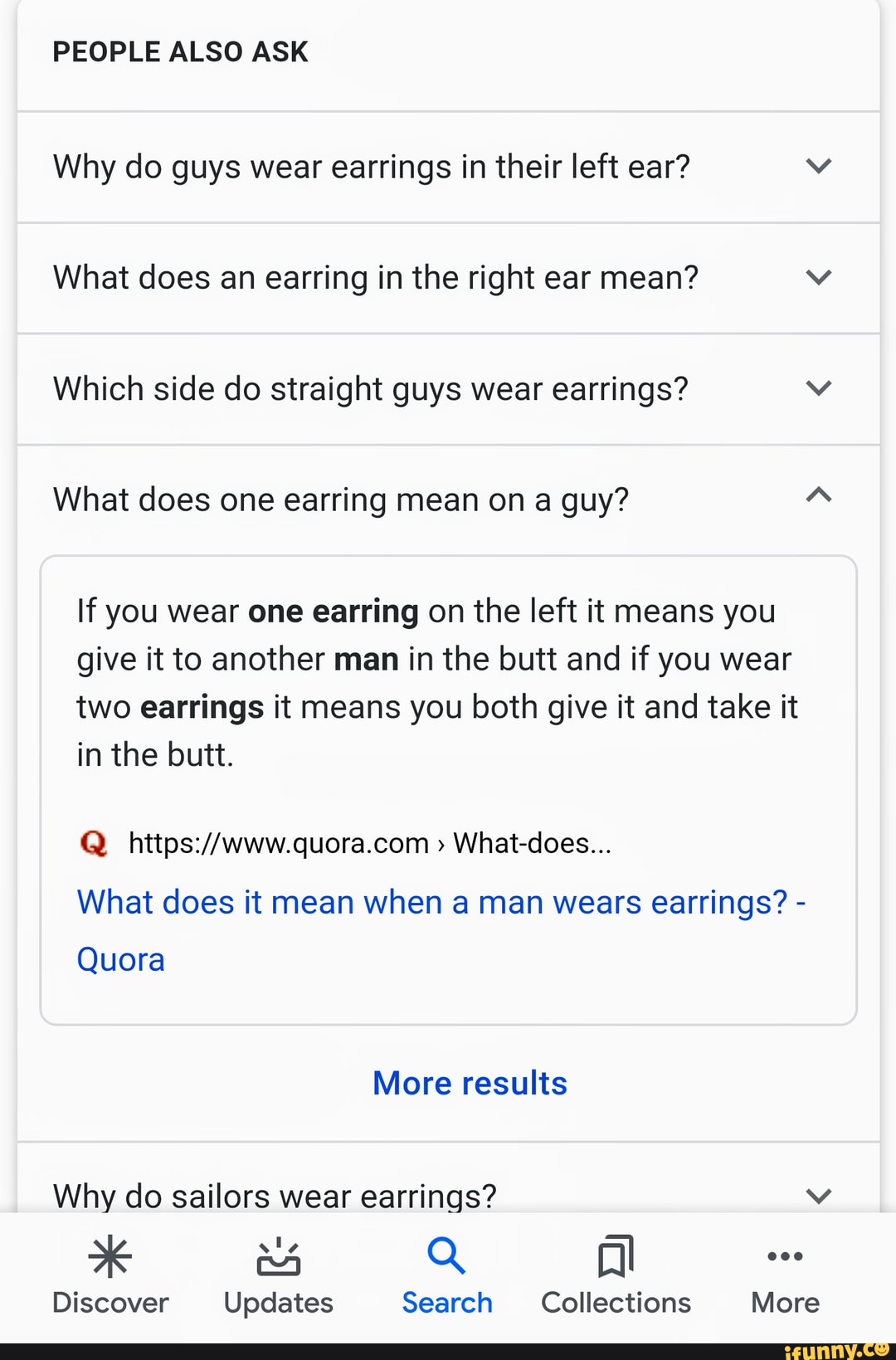This photograph showcases a set of online search results presented in a portrait-oriented format, which is notably taller than it is wide—almost twice as tall. The image is framed against a gray background, featuring a shadow effect on the left and right edges. 

At the very top of the image, partially cut off, is a black header that reads "People also ask." Following this header are several horizontally separated sections containing different text queries. The first query is presented in a long, horizontal box with the text, "Why do guys wear earrings in their left ear?" accompanied by a drop-down caret. Below this, another query reads, "Why does an earring in the right ear mean?" with a similar drop-down caret.

Continuing down, the next question is, "Which side do straight guys wear earrings?" also followed by a drop-down caret. This is succeeded by the query, "What does one earring mean on a guy?" which features an upward caret indicating an expanded answer. The provided result in the text box poses a controversial and explicit statement: "If you wear one earring on the left, it means you give it to another man in the butt. And if you wear two earrings, it means you both give it and take it in the butt." 

To the left of this text box is a red "Q" logo, suggesting the source is qora.com. Following this is a hyperlink to the website, displayed in blue. Below the text box, a blue link reads "More results."

At the bottom of the image, another query, "Why do sealers wear earrings?" is shown in a similar styled box. The footer section of the image contains navigational options, including Discover, Updates, Search, Collections, and More, with the "Search" option highlighted by a blue magnifying glass icon.